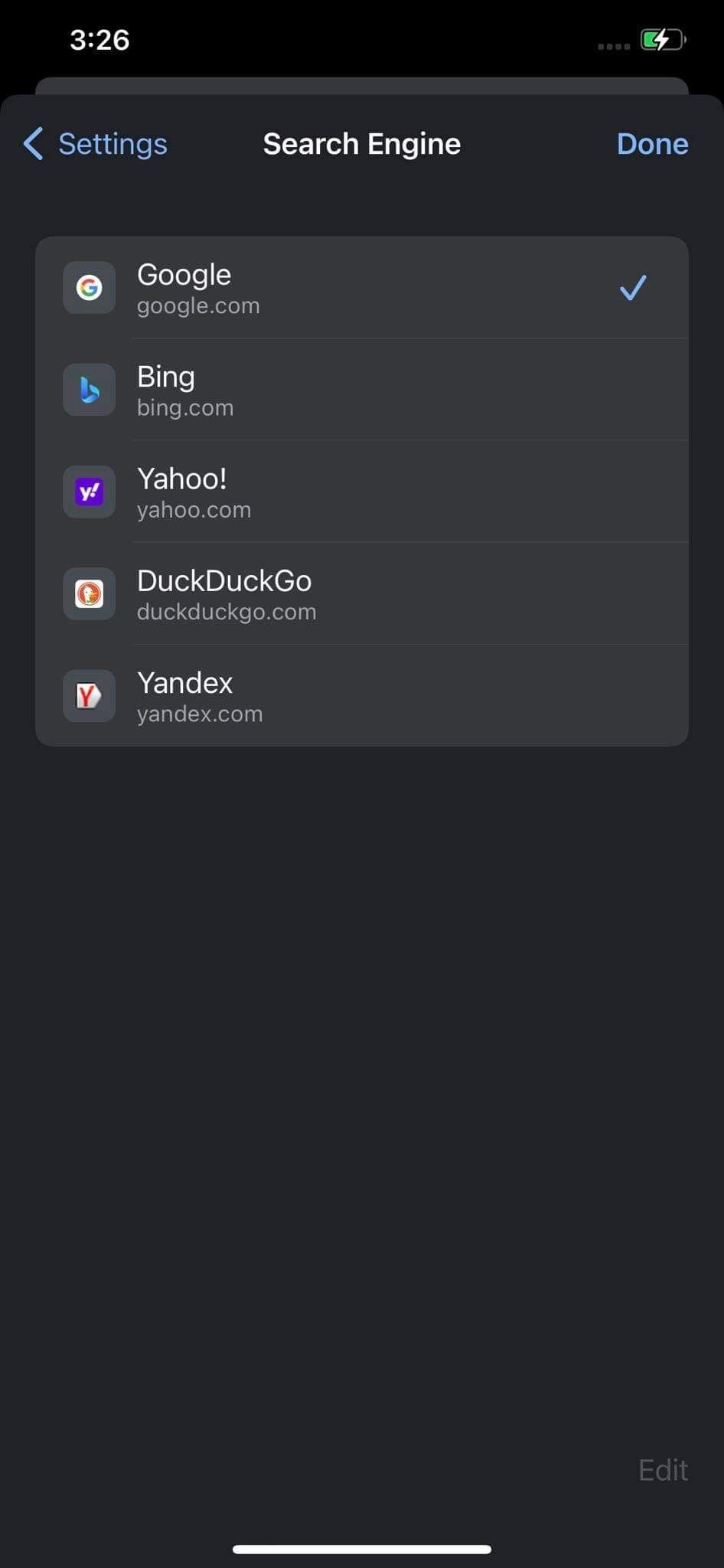The image shows a black screen with a digital clock displaying the time "3:26" at the top. Directly below the time, the word "Settings" is displayed in pale blue, accompanied by a left-pointing arrow. To the right of this text, there is a pale blue button labeled "Done." It is unclear whether this button is currently highlighted due to its light coloration.

Beneath this section, there is a list of search engines. At the top of the list, "Google" is displayed with the Google logo to the left and "google.com" noted beside it. This option is marked with a checkmark, indicating it is the selected search engine. 

Following Google, the list includes "bing.com" with the Bing logo, "yahoo.com" with the Yahoo logo, "duckduckgo.com" with the DuckDuckGo logo, and lastly "yandex.com" with the Yandex logo. Each search engine name and URL is accompanied by its respective logo on the left. The user remarks that while they are familiar with Google, Bing, Yahoo, and DuckDuckGo, they are not familiar with Yandex, and they note that all entries appear to be search engines.